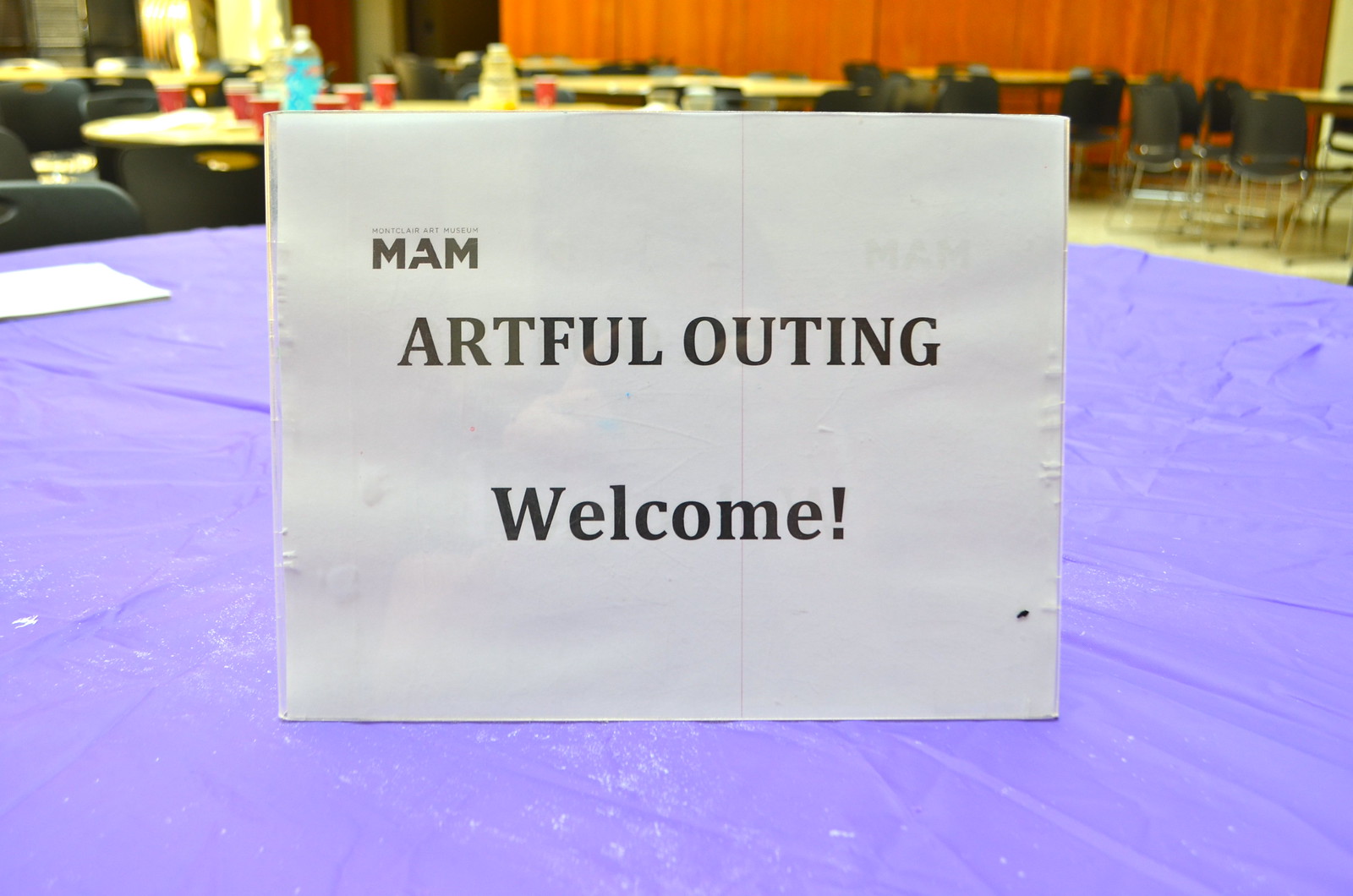This image depicts a round table covered with a lavender tablecloth, centrally adorned with a white sign featuring black lettering. The sign reads "MAM Artful Outing Welcome," suggesting a warm greeting for attendees at what appears to be a conference or get-together. The venue is an indoor setting with other seating arrangements visible in the background. Surrounding tables are draped in various colored tablecloths, some with red cups and additional items indicative of a gathering. Black chairs are arranged around these tables, and elements such as an orange curtain and lighting fixtures are present, enhancing the venue’s ambiance. Notable details include bottles with blue and yellow labels containing clear, yellow, and black liquids, suggesting beverages provided for the event. The overall scene suggests a well-organized event in a public or institutional setting, like a school or community center.